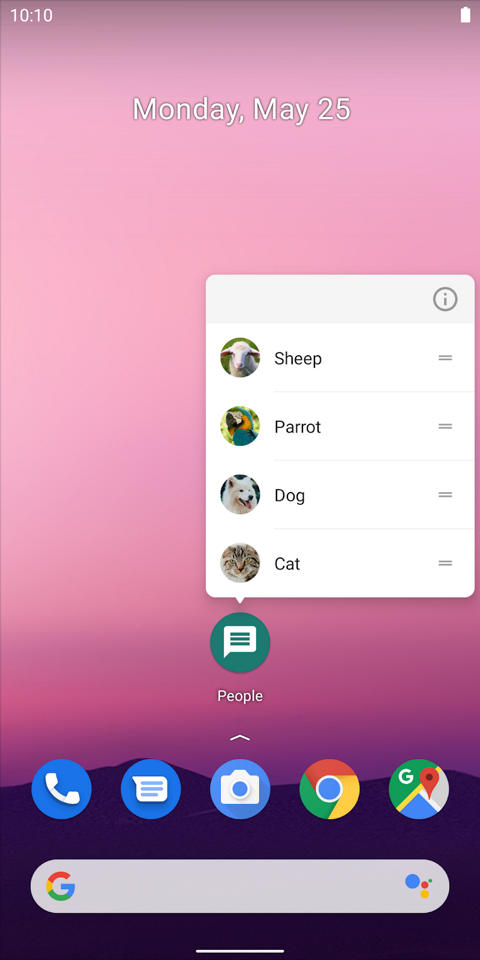A mobile device screenshot features a beautifully vibrant gradient background, transitioning from dark pink at the top, to a lighter pink in the center, and back to dark pink at the bottom, culminating in a black silhouette of a mountain range at the bottom of the screen. 

At the very top of the display, the time is shown in white as "10:10," accompanied by a battery icon on the far right. Below the time, the date "Monday, May 25th" is prominently displayed in white lettering.

The home screen includes several visual elements. A green box with a white text box in its middle, currently selected, sits near the top. Adjacent to this is a white box with a gray top, featuring selectable options labeled "Sheep," "Parrot," "Dog," and "Cat."

Beneath these options, a horizontal row of icons is arranged as follows: a purple phone icon with a white phone symbol, a purple bubble with a text messaging symbol, a blue bubble with a camera symbol, the Google Chrome logo, and the Google Maps logo.

Below this row, a gray search box with the colorful 'G' Google logo on the left and an unfamiliar icon on the right is displayed. At the very bottom of the screen is a gray bar indicating the swipe-up gesture for access to additional functionalities.